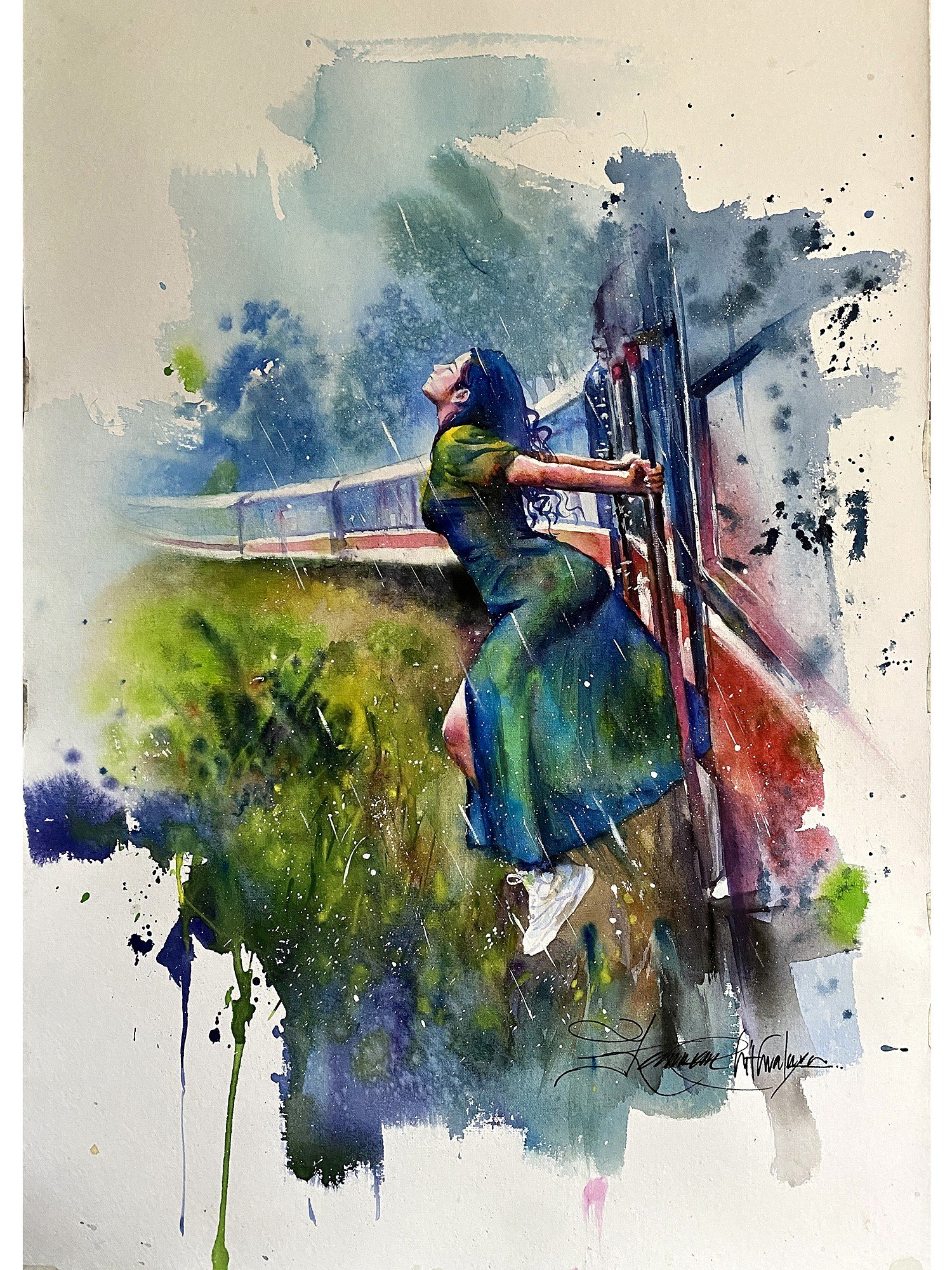This rectangular watercolor painting, approximately five to six inches high and four inches wide, depicts a striking, semi-realistic scene of a woman leaning out of a train. The background transitions from a light brown at the top to a light gray and off-white towards the bottom, while green foliage and blue highlights frame the lower section. The woman, who has light brown skin and black hair, is captured hanging out of a white railcar with red stripes, her back arched forward and her head tilted upward toward the sky. She is holding onto two railings with her arms extended behind her. Dressed in a clinging green, blue, and yellow dress, she appears wet from the rain, which is suggested by blue-green droplets descending around her. Her white sneakers and the tip of one knee are visible through the soaked fabric. The scene evokes a sense of serene embrace of the rain and nature around her, reinforced by the surrounding green trees and the train's path. The painting bears a signature in the bottom right corner, hinting at its status as a carefully scanned and preserved artwork, possibly created on notebook paper, given its subtle staple markings and worn edges.